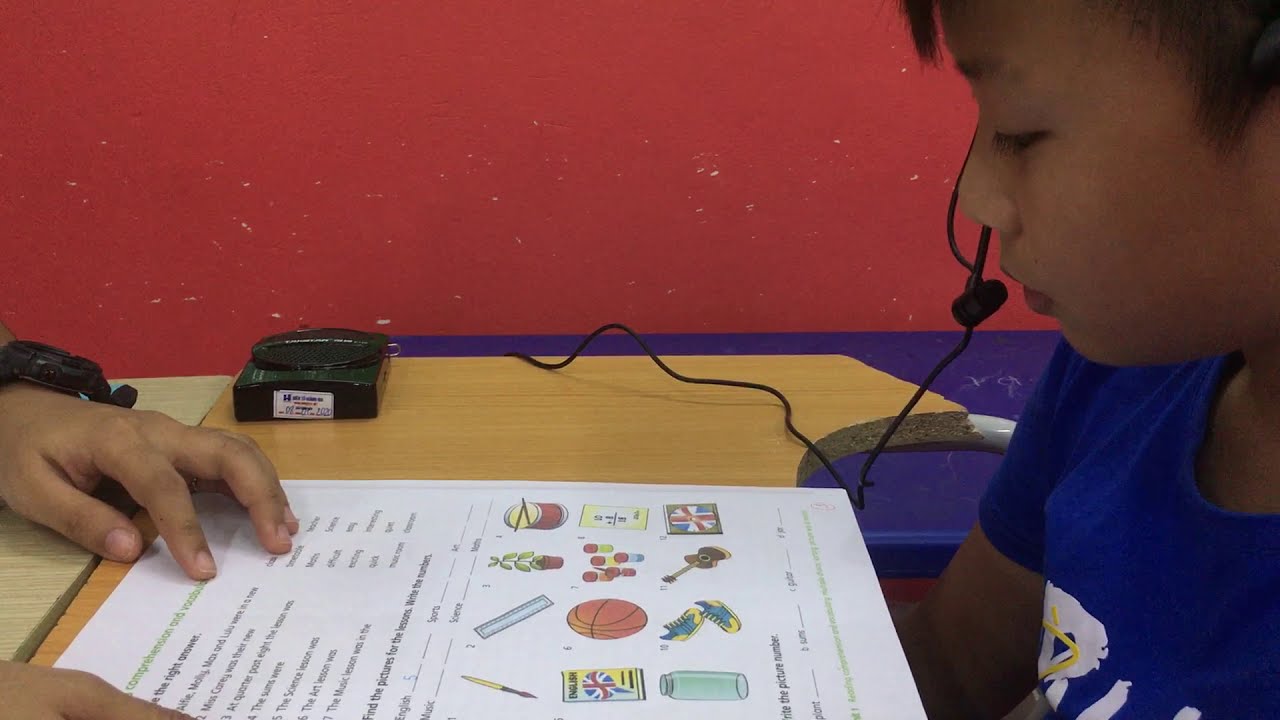The image features a close-up of a young boy, approximately eight or nine years old, seated at a light-colored desk. He is wearing a blue short-sleeved t-shirt with white lettering. The boy, who appears to be of Asian descent, has a headset with a small microphone on, and a wire trailing from it, which is attached to a small square device resembling a tape recorder on the desk. The boy's dark hair and his focused downward gaze are visible, as he looks at a colorful worksheet on the desk. This worksheet includes pictures of a basketball, a guitar, sneakers, a ruler, and other items, with some words and fill-in-the-blank sections. The teacher is present in the frame, though only their hands are visible; the left hand, sporting a watch, points to the worksheet, guiding the student. In the background, there are hints of a blue table and a prominent red wall.